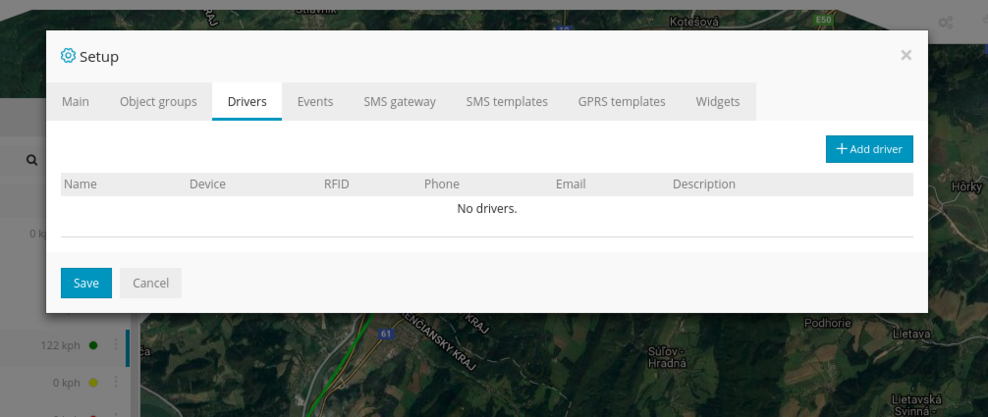The image is a screenshot of a web page featuring a map in the background that displays roads and street signs. Overlaid on the map is a prominent text box. In the upper left-hand corner of the text box, a blue sprocket icon is accompanied by the black text "Set Up." The upper right-hand corner of the text box features a gray 'X' icon for closing the window.

Directly below, the text box is filled with several horizontally aligned gray boxes, each with a distinct header. Among these headers, "Main Objective Groups," "Drivers," "Events," "SMS Gateway," "SMS Templates," "GPRS Templates," and "Widgets" are listed in dark gray text against a gray background. Notably, the "Drivers" header stands out with white text and a blue underline.

Further down, another bar with a light gray background and dark gray text is visible, listing columns titled "Names," "Device," "RFID," "Phone," "Email," and "Description." On the far right of this bar, a blue button with white text reads "+ Add Driver."

In the center of the text box, the phrase "No Drivers" is displayed in black text, indicating the absence of any driver entries. Finally, in the lower left-hand corner of the text box, there are two buttons: a "Save" button with a blue background and white text, and a "Cancel" button with a light gray background and dark gray text.